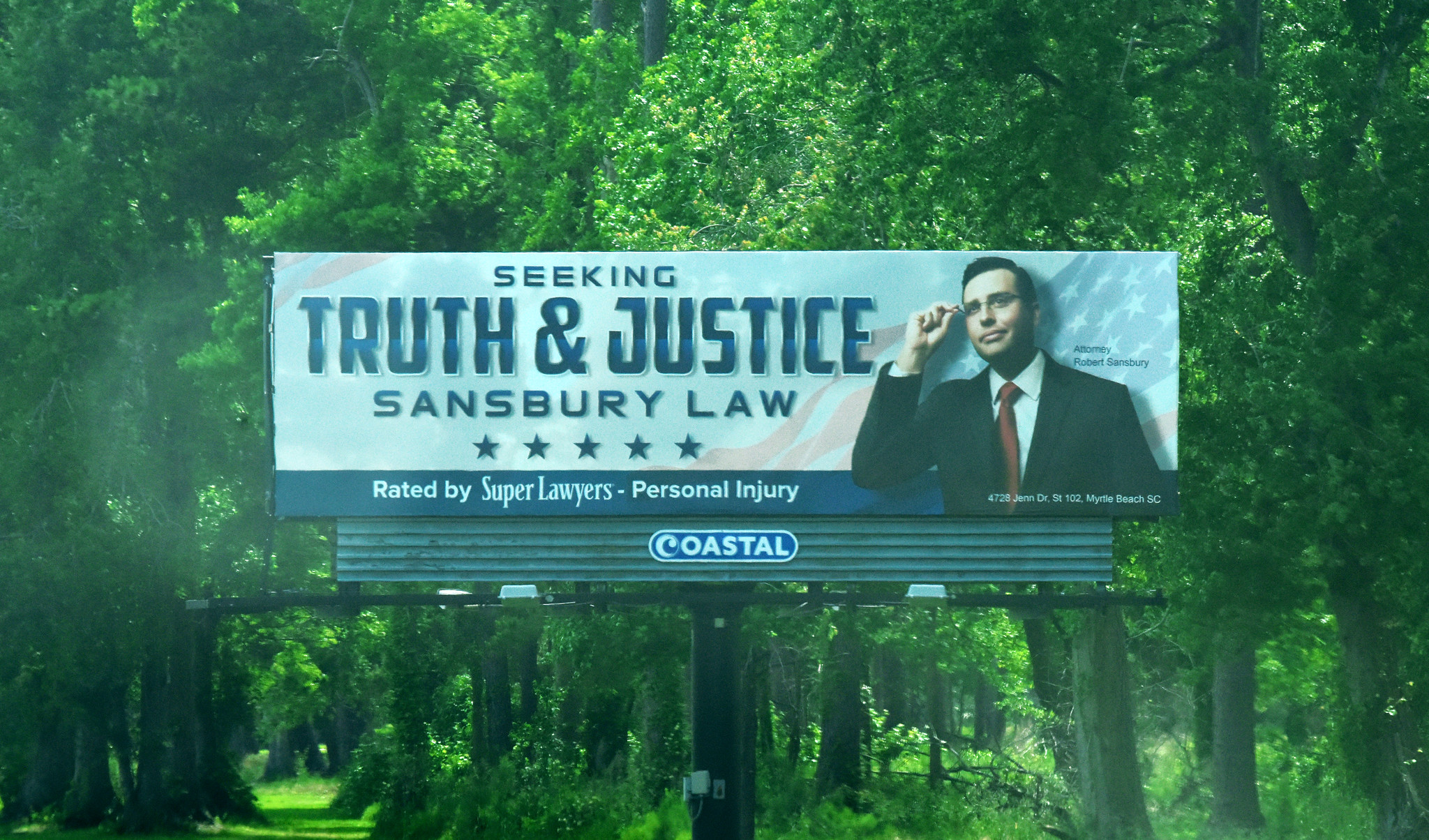A rectangular billboard stands prominently against a backdrop of thickly planted trees with dense, overlapping green leaves. The trees are interspersed with patches of grass, creating a lush, wooded scene. The photograph appears to be taken through a windshield, casting a bluish-green hue over the entire image. 

The billboard itself is long and not very tall, mounted on a single metal tubular post with a black frame. It features a distinguished gentleman who is holding his glasses with his right finger and thumb. He is dressed in a suit and tie, with a red tie and a white shirt, exuding an air of professionalism. Beside him, the billboard text reads "Attorney Robert Saxbury," with the gentleman standing against a background of a faint American flag billowing in the wind.

On the left-hand side of the billboard, in blue or gray text, the inspirational slogan "Seeking Truth and Justice" is displayed, followed by "Saxbury Law." Along the bottom of the billboard, it emphasizes the lawyer’s credentials, stating "Rated by Super Lawyers, Personal Injury." The contact information provided is for an office located at Jen Drive Street, Suite 102, in Myrtle Beach, South Carolina.